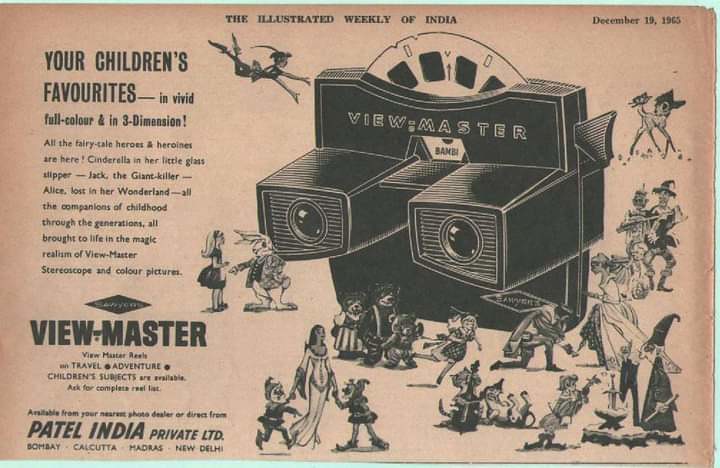This advertisement from the Illustrated Weekly of India, dated December 19, 1965, showcases the View-Master stereoscope. The ad, printed on faded maroon paper with black ink, features a striking View-Master gadget, predominantly black in color with the 'View-Master' logo prominently displayed. Centered in the gadget is a circular white reel holder with squares inside, containing the word 'Bambi'. This innovative gadget is designed to display vivid full-color 3D images of beloved characters from classic fairy tales and Disney movies. Surrounding the gadget in the ad are whimsical illustrations of these cherished characters, including Cinderella in her glass slipper, Alice from Wonderland, Bambi, Peter Pan, and others like Robin Hood and Snow White and the Seven Dwarfs. On the left side of the advertisement, text in bold letters announces: "Your children's favorites in vivid full color and in 3D dimension. All the fairytale heroes and heroines are here, brought to life in the magic realism of View-Master stereoscope and color pictures." Below this message, additional details encourage customers to ask for a complete list of View-Master reels, available from their nearest photo dealer or directly from Patel India Private Ltd. in Bombay, Calcutta, Madras, and New Delhi.